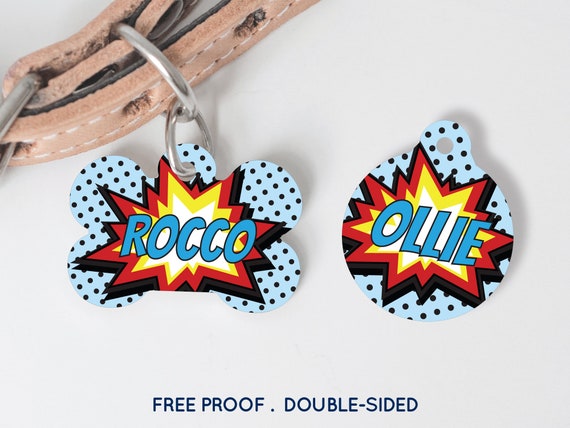This detailed color photograph, captured indoors in a landscape orientation, showcases two distinct pet tags prominently centered within the frame. The left tag is bone-shaped and attached to a silver D-ring on a beige leash. It features a light blue background with black polka dots. At the center of this tag is a vibrant starburst pattern radiating outwards in white, yellow, red, and black. The name "Rocco" is boldly inscribed across the starburst in bright blue font with a black outline. The adjacent tag on the right is circular, mimicking a Christmas ornament. It displays a matching light blue and black polka dot background and a similar starburst design. "Ollie" is written at its center in the same striking blue font. The base of the image has a light gray background with the words "FREE PROOF DOUBLE SIDED" clearly printed in capital letters using a navy blue sans-serif font. The photograph is approximately four inches wide and three inches high, set against a minimalistic and sleek grey background, emphasizing the product photography's realistic and detailed nature.